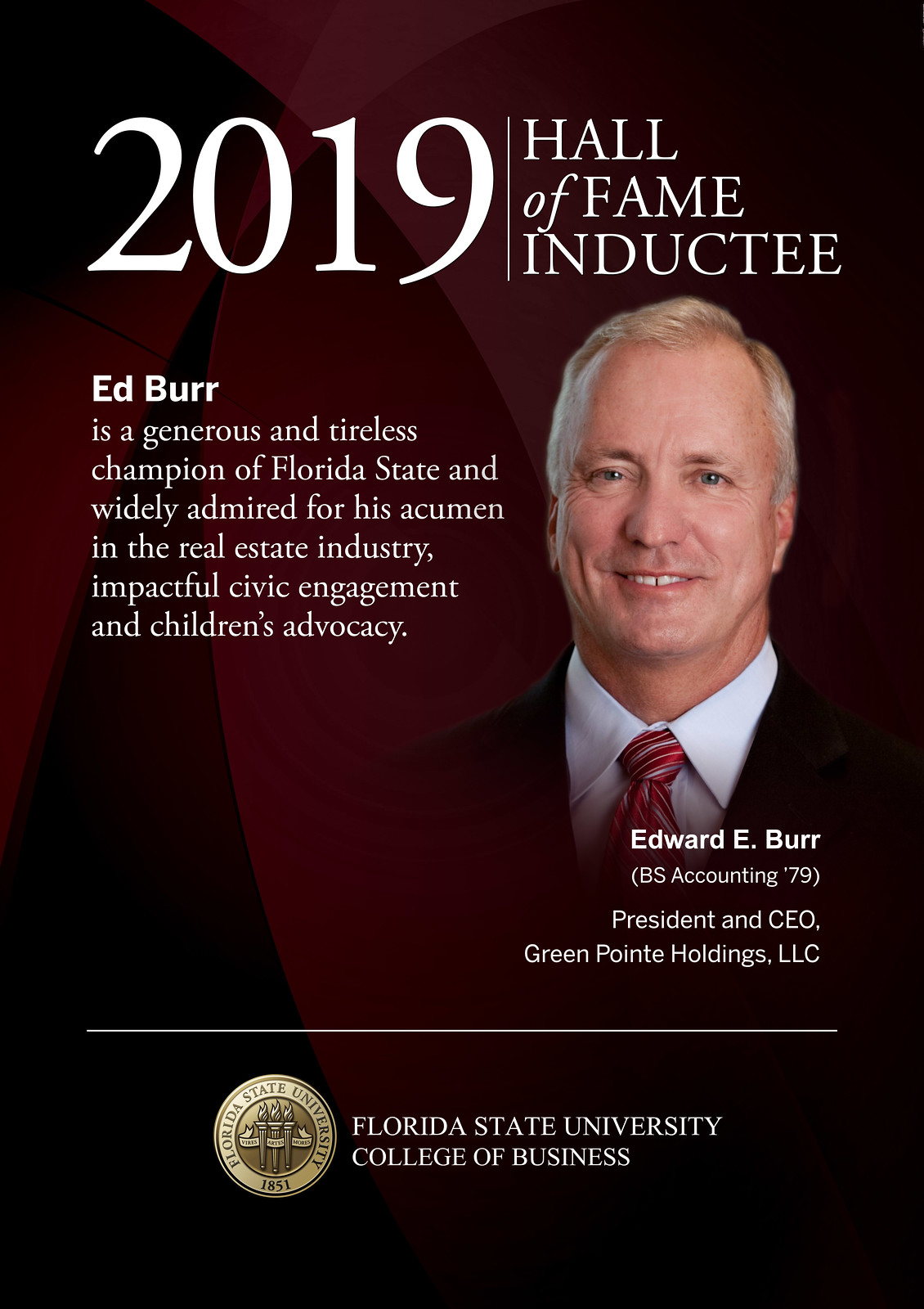The image features an informational sign highlighting Edward E. Burr, President and CEO of Greenpoint Holdings, LLC, who was inducted into the Florida State University College of Business Hall of Fame in 2019. The sign has a black background with white lettering and a gold emblem of Florida State University. 

At the top of the image, "2019 Hall of Fame Inductee" is prominently displayed. Below this title, a detailed description reads: "Ed Burr is a generous and tireless champion of Florida State, widely admired for his acumen in the real estate industry, impactful civic engagement, and children's advocacy."

A large photograph of Ed Burr is situated on the right side of the sign. Burr has short brown hair, blue eyes, thin brown eyebrows, and a slight smile, revealing a small gap in his teeth. He is dressed in a black suit, white dress shirt, and a red tie with silver stripes.

Below the photograph, additional text states: "Edward E. Burr, BS Accounting '79, President and CEO, Greenpoint Holdings, LLC."